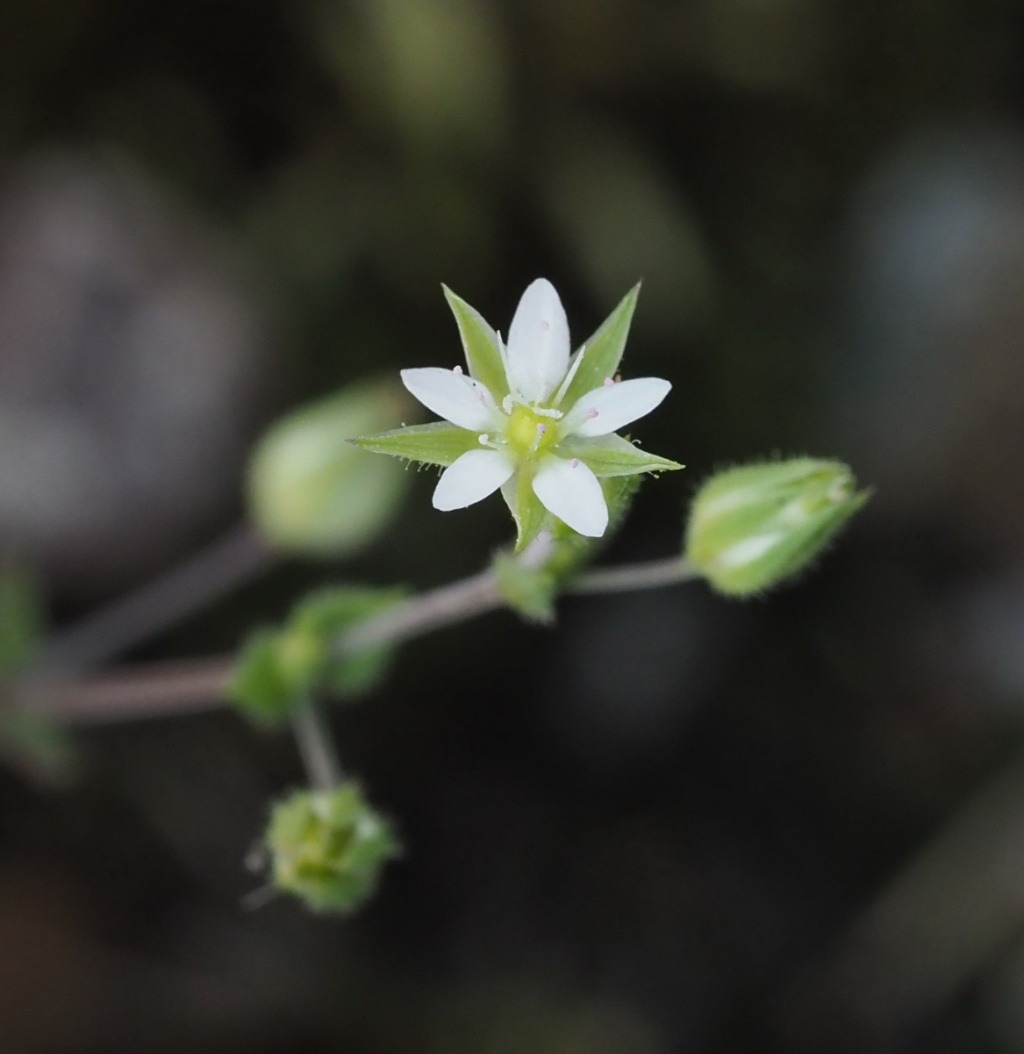A captivating close-up outdoor photograph centers on a delicate white flower in full bloom. The flower, approximately the size of a quarter, features five white, rounded petals and light green leaves. At its center, a yellowish region with a hint of green stands prominently, surrounded by slender white stems. The flower is attached to a light purple stem, which runs diagonally from the middle left towards the upper right of the frame. The foreground is clear, placing emphasis on the flower, while two unopened green pods flank it in the blurred background. The entire backdrop is a deep, indistinct shade, likely indicating a shaded area, accentuating the vivid details of the blossom.